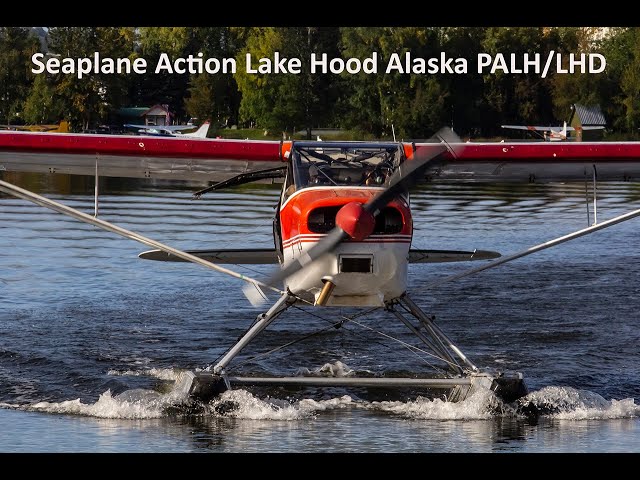This detailed photograph captures the front view of a seaplane either landing or taking off from the water at Lake Hood, Alaska. The seaplane, predominantly white with striking red accents on the top and on its wings, is equipped with a black propeller whose center is red and is either starting to spin or slowing down, as suggested by the visible shadow. You can also notice silver metal supports crisscrossing at the front, holding the plane's boat-like floats on the water, causing small ripples. The seaplane is framed centrally in the image, and the wings are partially cropped out. In the backdrop, the shoreline is dotted with several docked seaplanes, houses, and a forested area. The scene bathes in daylight under a clear, bright sky. At the top, the caption in white text reads, "Seaplane Action, Lake Hood, Alaska, PALH-LHD."